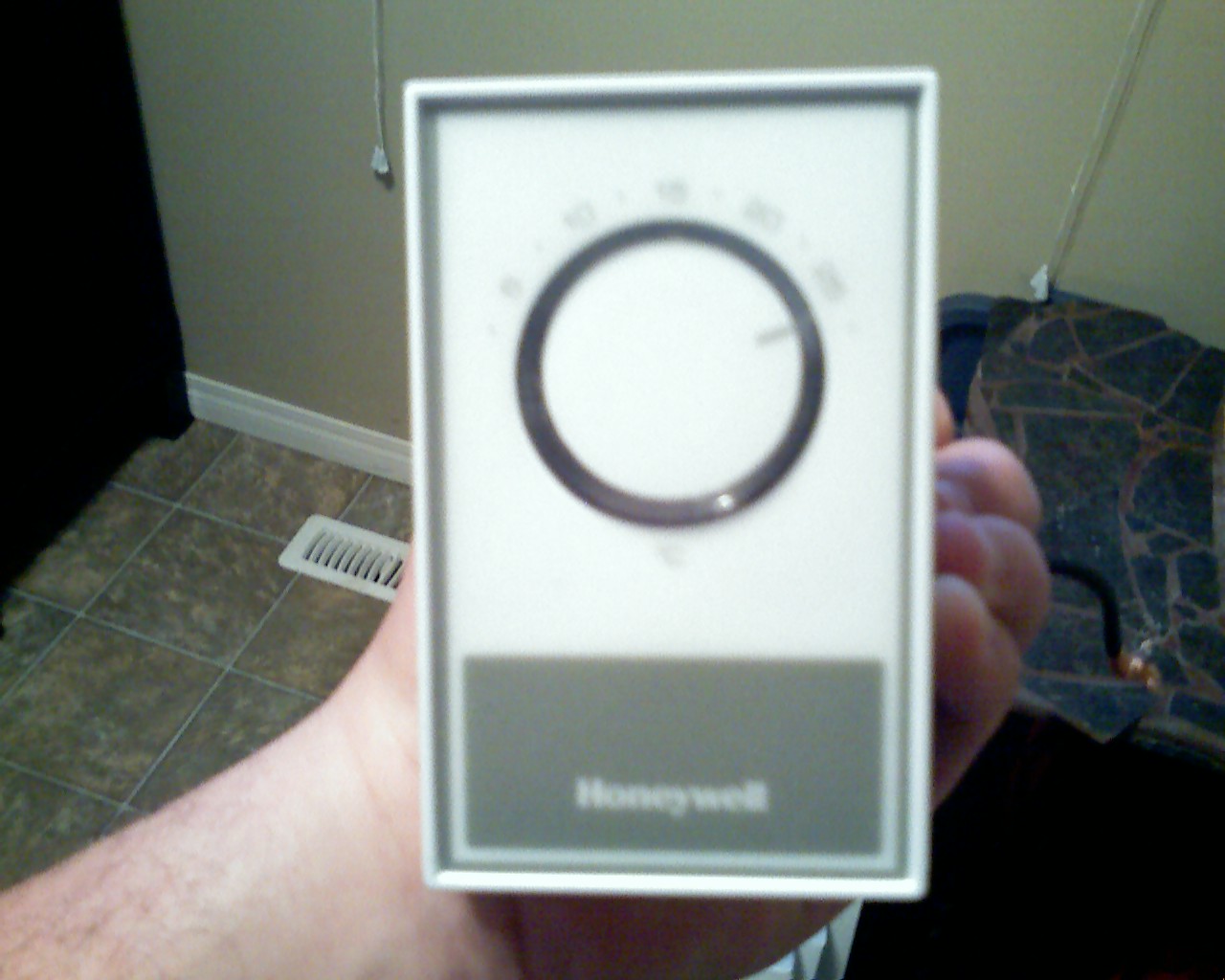A slightly blurry indoor photograph captures the interior of a house or apartment. The beige wall adorned with white trim is a prominent feature, above a floor covered in brown and gray tiles. A white floor register for heating and cooling is embedded in the floor. In the left-hand side of the image, partially visible and out of focus, is a blue piece of furniture, potentially a couch or chair. The foreground showcases a hand holding an analog, dial-based thermostat, characterized by its square, white housing with a gray bottom section. The thermostat, bearing the brand name "Honeywell," lacks any digital buttons or screens, emphasizing its vintage design.